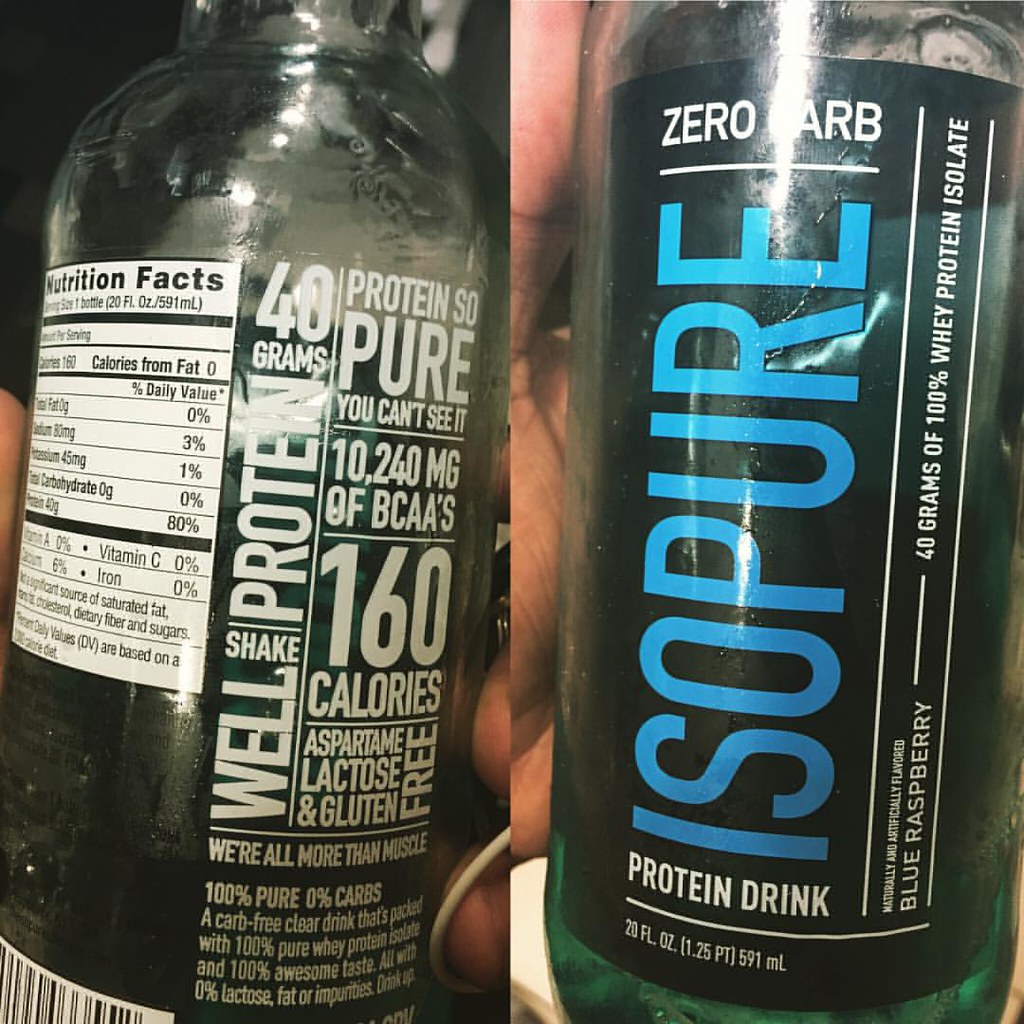This image consists of two photos showcasing different sides of a single clear glass bottle of Isopure protein drink. On the right photo, the front label prominently features the word "Isopure" in large blue letters running vertically, with "zero carb" positioned above it. Below, in white text, it reads "protein drink," specifying "24 ounces, 1.25 pt, 591 ml." Further down the label, the drink is described as "blue raspberry" flavored and containing "40 grams of 100% whey protein isolate," with a note indicating it is "naturally and artificially flavored." The left photo displays the back of the bottle, which includes a white "Shake Well" instruction and detailed nutritional information in black text on a white background. Key highlights include "40 grams Protein, protein so pure you can't see it," "10,240 mg of BCAAs," "160 calories," and "aspartame, lactose, and gluten free." The label also underscores that it's a "carb free clear drink" with "100% pure whey protein isolate" and boasts "100% awesome taste, 0% lactose, fat, or impurities." Both photos have a human hand partially visible behind the bottles, and the nutrition facts are partially obscured.